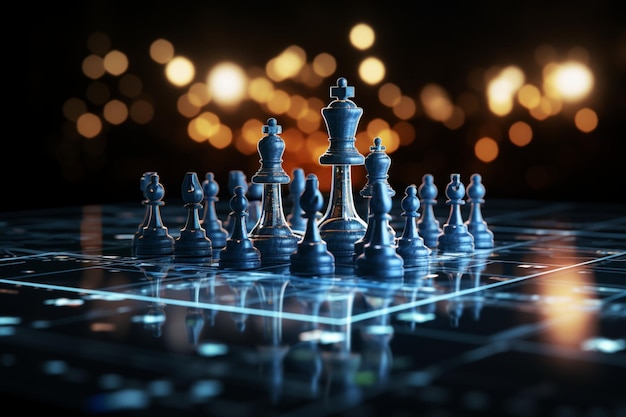In this detailed image, we see a modern, reflective chessboard set against a dark background. The chessboard itself has a black base with striking blue lines and details, giving it a contemporary and glassy appearance. There are various chess pieces, including the king, queen, bishop, rook, knight, and pawns, all rendered in a light blue color. The tallest piece, the king, stands prominently in the center, flanked by smaller pieces. The pieces are sharply in focus, allowing their intricate details to be clearly visible. Behind the chess set, the background is blurred and features numerous circles of light in hues of orange, yellow, and white. These vivid, glowing lights create a dramatic contrast against the black background, illuminating the chess pieces and giving them a luminous, almost ethereal aura. The entire scene is viewed from a frontal perspective, showcasing the reflection of the chess pieces on the glossy surface of the chessboard, adding to the image's overall depth and visual appeal.